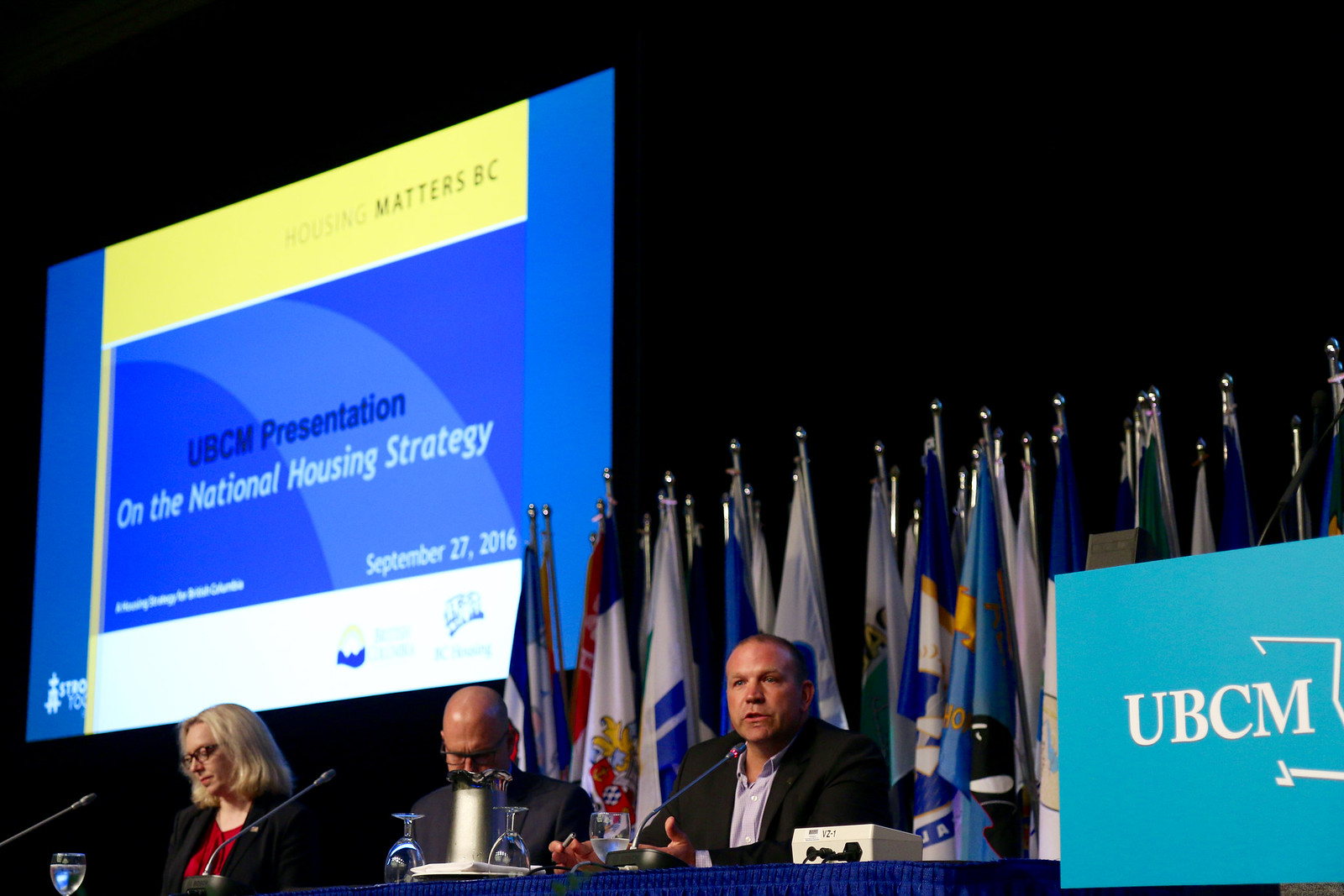Three individuals are seated at a desk on a stage, set against a backdrop of multiple flags on flagpoles. In the center is a man with brown hair, wearing a black jacket over a blue button-up shirt. His face, slightly red and glistening with light reflected off his forehead, is directed straight forward as he holds his hands in front with a thumbs up gesture. A microphone is positioned near his chin. To his right is a bald man in a black suit, looking downwards. To the left is a woman with blonde hair just below her ears, wearing dark glasses, a black jacket, and a red shirt, staring downward and to the left. In front of them on the desk, several glasses can be seen, one of which appears to contain a beverage.

Above them, an illuminated square projection displays the title "UBCM Presentation," set within dark blue and yellow sections. The text "Housing Matters BC" is prominently featured at the top, with additional details about the National Housing Strategy and the date, September 27, 2016, visible below. A teal square in the bottom right corner bears the UBCM logo in white letters.

A podium with the white UBCM logo against an aqua blue background stands in the foreground. The overall setting, characterized by its professional ambiance, flags, and detailed presentation slide, indicates that the photograph was taken during a conference focused on housing strategies.